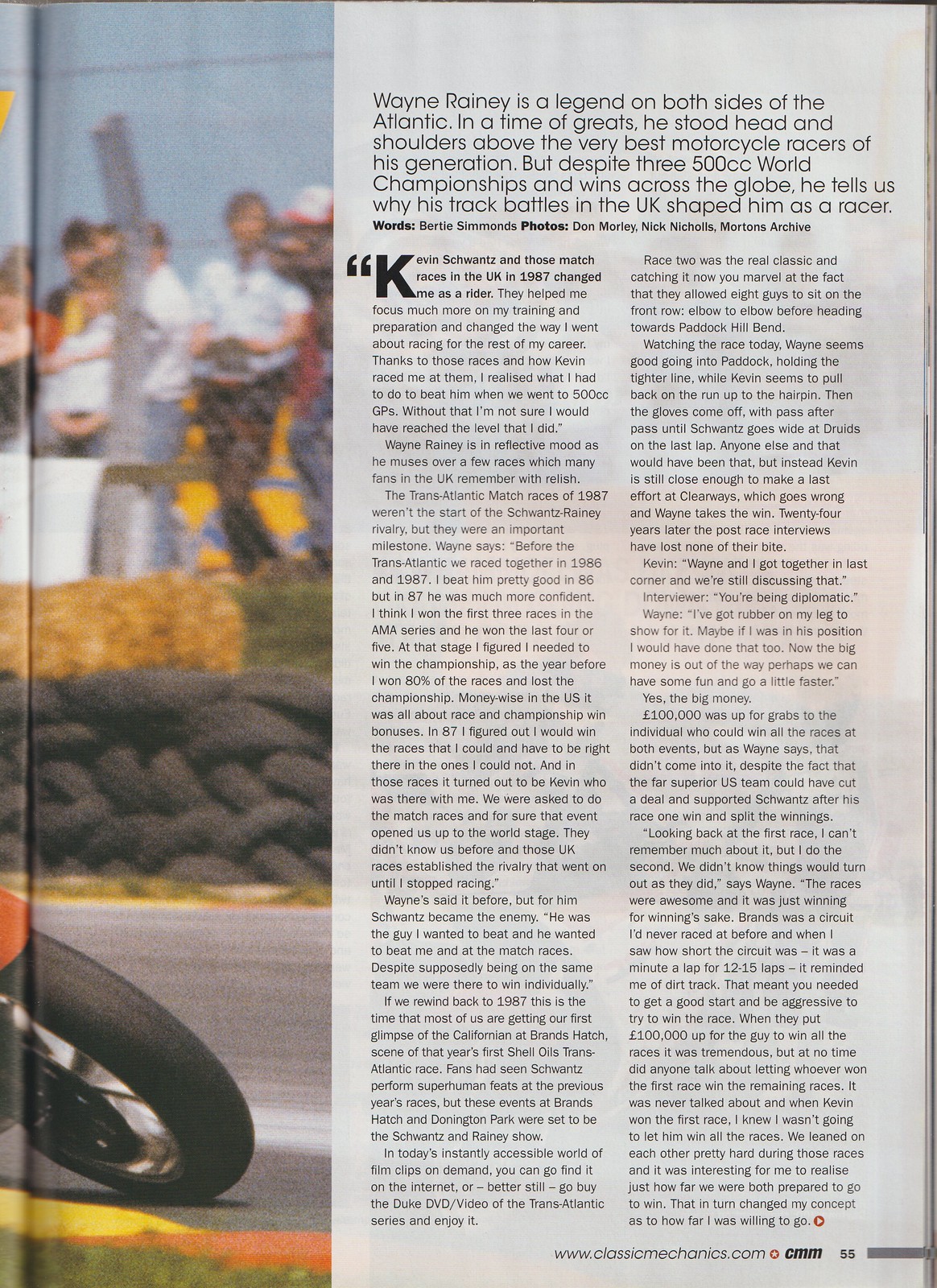The inside page of the magazine, open to page 55, is divided into three distinct sections. Near the spine, the left column showcases a vertical image spanning from the top to the bottom of the page. This image depicts a motorcycle racecourse scene with a blurred, sky-blue background, people standing behind a fence, hay bales, numerous black tires, a road, some grass, and part of a motorcycle wheel visible in the foreground. The remaining two-thirds of the page is dedicated to a full-length article on a white background with fine black print. The article begins prominently with the paragraph: "Wayne Rainey is a legend on both sides of the Atlantic. In a time of greats, he stood head and shoulders above the very best motorcycle racers of his generation. Despite three 500cc world championships and wins across the globe, he tells us why his track battles in the UK shaped his career."